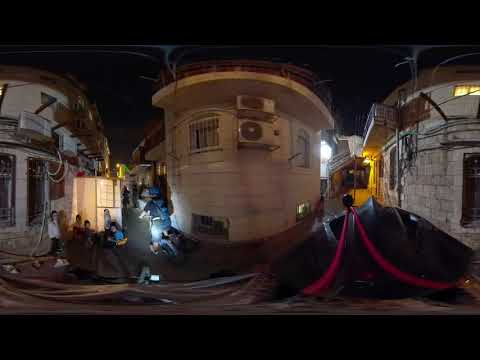The image depicts an outdoor nighttime scene with a panoramic view of three run-down, two-story white buildings. These buildings, likely made of stone or concrete blocks, appear rounded due to the lens distortion. They feature windows with bars and air conditioners installed at the top. The buildings look like they could use a fresh coat of paint. On the street level, there's a big black tarp with red trim on the right side. The left side shows approximately eight blurry people, giving the impression they are sitting or standing on the ground. The street looks somewhat disturbed, possibly indicating a movie set. The sky above is pitch black, adding to the nighttime atmosphere.